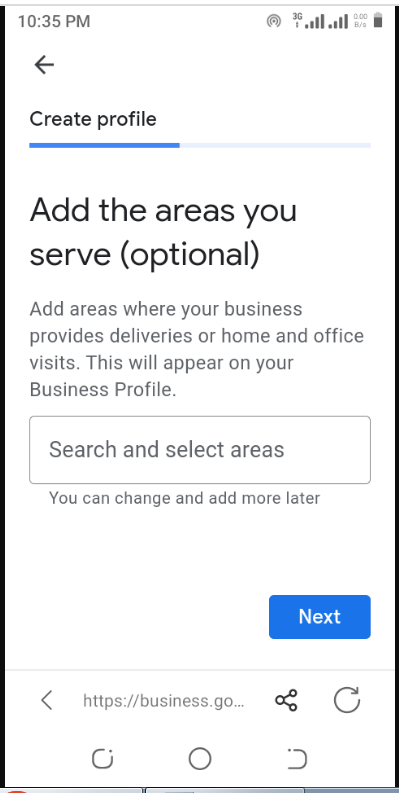The image depicts a smartphone screen displaying a user interface for creating a business profile. At the top of the screen, the time is displayed as "10:35 PM," alongside various standard icons like cellular signal strength and battery percentage. Below this, a gray back arrow is visible next to the text "Create Profile," and a blue progress bar indicating that the setup is about halfway complete.

The main section of the screen prompts the user to "Add the areas you serve," with a note in parentheses indicating that this step is optional. Beneath this prompt, gray text provides further guidance: "Add areas where your business provides deliveries or home and office visits. This will appear on your business profile." There is a search box labeled "Search and select areas" with an additional note that changes and additions can be made later.

The interface includes a prominent blue "Next" button to proceed with the setup. At the bottom of the screen, an incomplete URL "https://business.go" is displayed, accompanied by a refresh icon and a share button. Additionally, three navigation buttons are located at the bottom: a half-filled circle, a completely filled circle, and an open circle, all in black.

The background of the screen is predominantly white, featuring black and gray text, and the design elements are minimalistic but functional, focusing on user guidance for setting up the business profile.